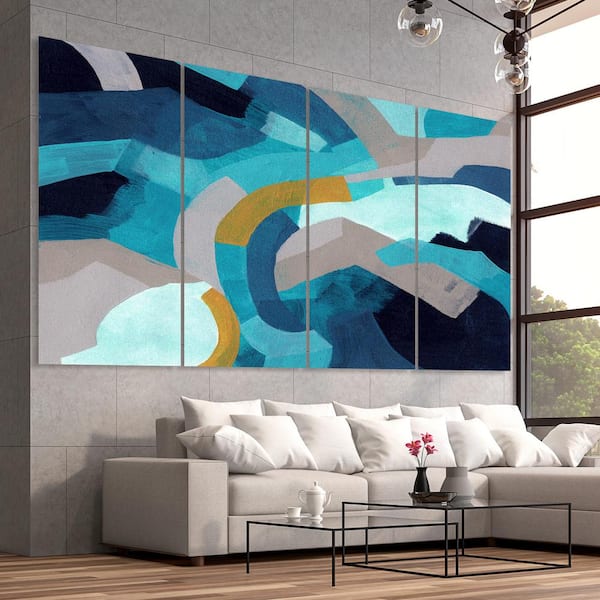The image depicts a modern, contemporary living room with a light and airy ambiance. The focal point is a sectional couch, primarily gray in color, adorned with an abundance of white throw pillows in two rows. The couch also features a chaise on the right side. Directly above the couch is a large, abstract canvas divided into four equal-sized panels, showcasing a swirling mix of colors—including dark blue, turquoise, gray, black, yellow, and light aqua—creating a dynamic visual interest against the gray tiled wall.

To the right of the living room are large windows with black trim, allowing ample natural light to flood the space and offering a view of a bright sky and green trees outside. The floor is adorned with light wood, adding warmth to the room.

In front of the couch are two glass coffee tables with black frames; the smaller table on the left holds a teapot and teacup, while the larger table on the right displays a black vase filled with pink flowers, a bowl, and an empty vase. Hanging from the ceiling are clear crystal lights suspended on black wires, contributing to the overall modern aesthetic. The space is impeccably lit, emphasizing the clean lines and contemporary décor throughout the room.